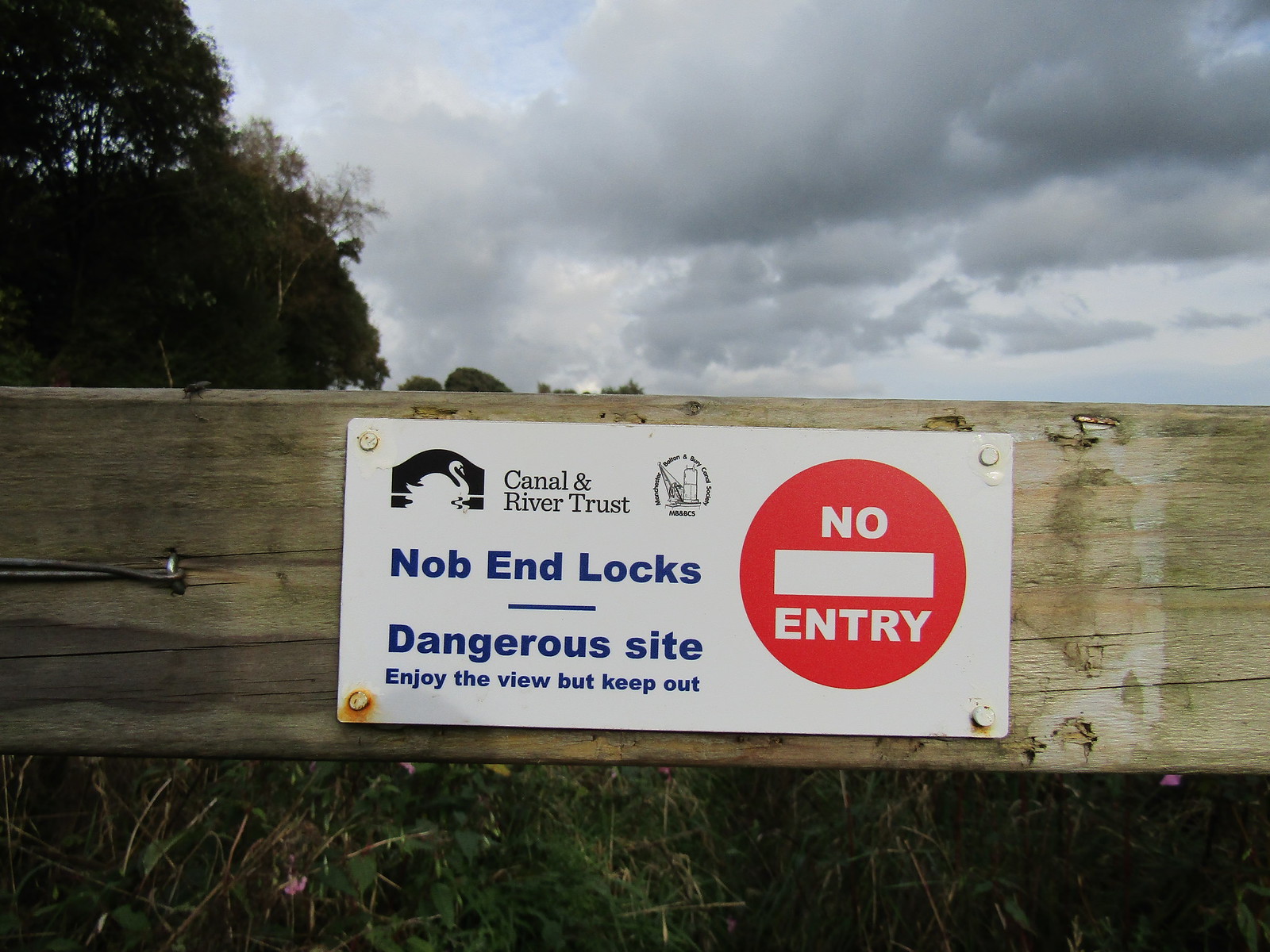This color photograph, taken outdoors, features a close-up of a white rectangular metal sign bolted onto a wooden fence. The fence and sign stretch across the center of the image. The sign's message reads: "Canal & River Trust. Knob End Locks. Dangerous Site. Enjoy the view, but keep out. No entry." The no entry warning is prominently displayed in white letters within a bright red circle. In the upper left corner of the sign, there's a swan-shaped logo representing the Canal & River Trust. Above the sign, the sky is filled with fluffy gray clouds, suggesting an overcast day that might lead to rain. To the left, tall, big green trees are visible, adding a natural frame to the scene. Below the sign, the ground is covered with green grass and dotted with purple flowers, looking slightly overgrown. Some bushes and additional greenery blur into the background.